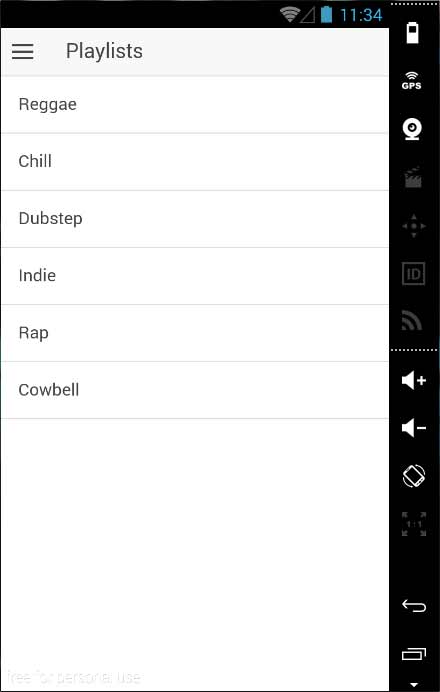This image is a screenshot of a phone displaying a list of playlists. The background of the screenshot is predominantly black, with a vertical white rectangle occupying the central portion. At the very top right edge of the rectangle, a series of status icons are visible: a gray Wi-Fi signal icon, cellular connection bars, a blue battery indicator, and blue text displaying the time "11:34". In the top right corner, a white battery icon is also present. Below these, there are several other icons including GPS signal, a moon icon indicating Do Not Disturb mode, a movie reel icon, an ID square, another Wi-Fi signal indicator, a volume up button, a volume down button, and a phone rotation icon.

Inside the white rectangle, at the top left corner, there are three lines stacked vertically, often representing a menu or "hamburger" icon. Beside this icon, the word "Playlists" is written in black text. Below this heading, several playlist names are listed vertically: "Reggae," "Chill," "Dubstep," "Indie," "Rap," and "Cowbell."